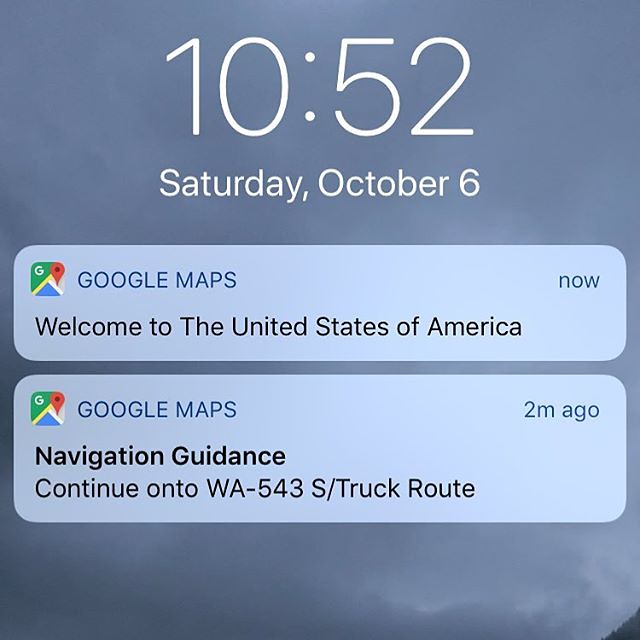A screenshot taken from an iPhone displays a cloudy sky-themed wallpaper with varying shades of blue and dark clouds. At the top, the time is shown as 10:52, with the date below reading Saturday, October 6. The screenshot reveals two Google Maps notifications. The first, marked 'Now,' welcomes the user to the United States of America. The second, received two minutes earlier, provides navigation guidance, instructing the user to continue on WA-543S/Truck Route.